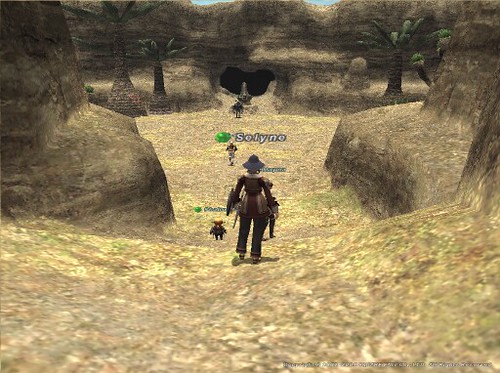This image is a detailed screenshot from a modern online video game, likely played on a PC or gaming console such as PlayStation or Xbox. The main character, prominently positioned in the center, is potentially named Solyne, identified by text above her head accompanied by a green dot. She wears a distinctive black bucket hat and is dressed in a brown long-sleeved shirt paired with dark-colored jeans or pants, giving her an appearance somewhat reminiscent of a scarecrow. Surrounding her is a brown, desolate landscape dominated by rugged mountains and rocky formations, with scattered trees that have green, cactus-like foliage. A shadow is faintly visible around her feet. In the foreground to her top left stands another character, partially obscured but also marked by a green dot and a readable name. Additional characters are present in the background, although they appear blurry or indistinct, with one notably short figure among them. Off-center towards the back, there is a prominent black opening, suggestive of a cave entrance, that adds to the scene's adventurous ambiance.